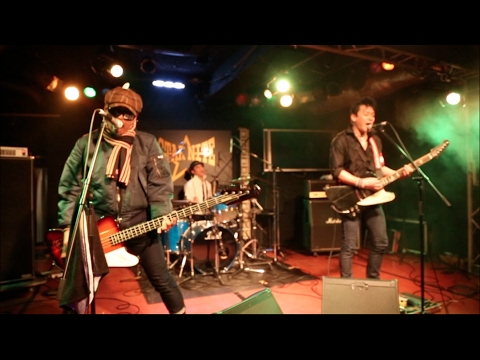The image captures a lively indoor concert featuring a three-man band on stage. The man on the left, who appears to be the bass player, stands in front of a microphone, gripping his two-tone guitar with its wooden brown and white body. He wears a distinctive brown beret with a plaid pattern, a green jacket (illuminated by stage lighting), black pants, and a scarf draped over his shoulders. His stance is slightly spread, and his guitar is held just below halfway down the neck. On the right, another musician with a black shirt and dark pants passionately sings into a microphone with his mouth wide open. He also holds a two-tone electric guitar—black and white. Behind them, the drummer, seated at a blue drum set adorned with a black bass drum, is seen energetically playing. Above, several bright stage lights in various colors (orange, green, white, neon blue, and yellow) illuminate the scene, casting dynamic shadows and reflections across the red ground and smoke-filled air. The backdrop features a screen with yellow writing, possibly the band's name, flanked by amplifiers and other equipment, contributing to the gritty, professional ambiance of the stage. The photo's fisheye effect adds a subtle curvature, immersing the viewer in the electrifying performance.